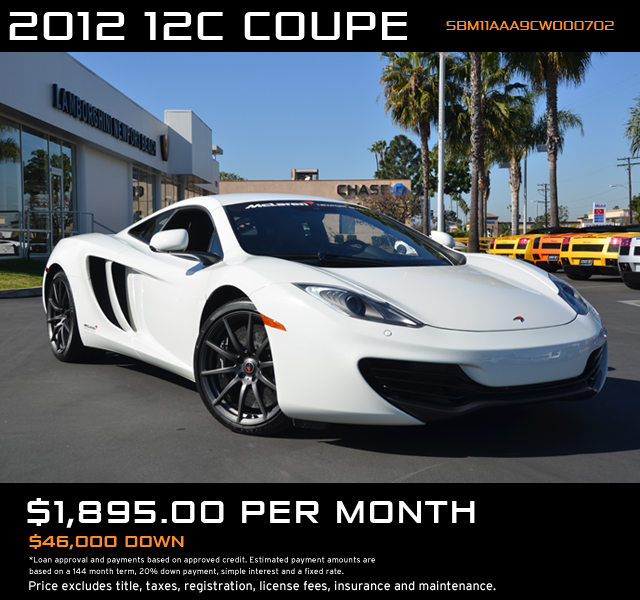The image features a white 2012 12C Coupe, prominently positioned diagonally in the center of the frame on an asphalt surface in an outdoor setting with bright, midday lighting. The car—potentially a Ferrari or Porsche—is characterized by its sloping windshield, black tires, deep recessed grille, and aggressive styling with side vents. Surrounding the main vehicle, there are several other cars in various colors including yellow and orange, all parked in a lot with a white dealership building to the left and a Chase Bank in the background, indicating a commercial area. Tropical palm trees are visible in the upper right corner, suggesting a temperate or tropical U.S. location. Overlaying the image, there are two black horizontal bands with white and gold text. The upper band reads "2012 12C Coupe" along with part of the VIN number, while the lower band states the financing details: "$18.95 per month," "$46,000 down," and notes about price exclusions regarding tax, title, registration, license fees, insurance, and maintenance. The overall style of the image is photographic realism, used here in what appears to be an advertisement for the car.